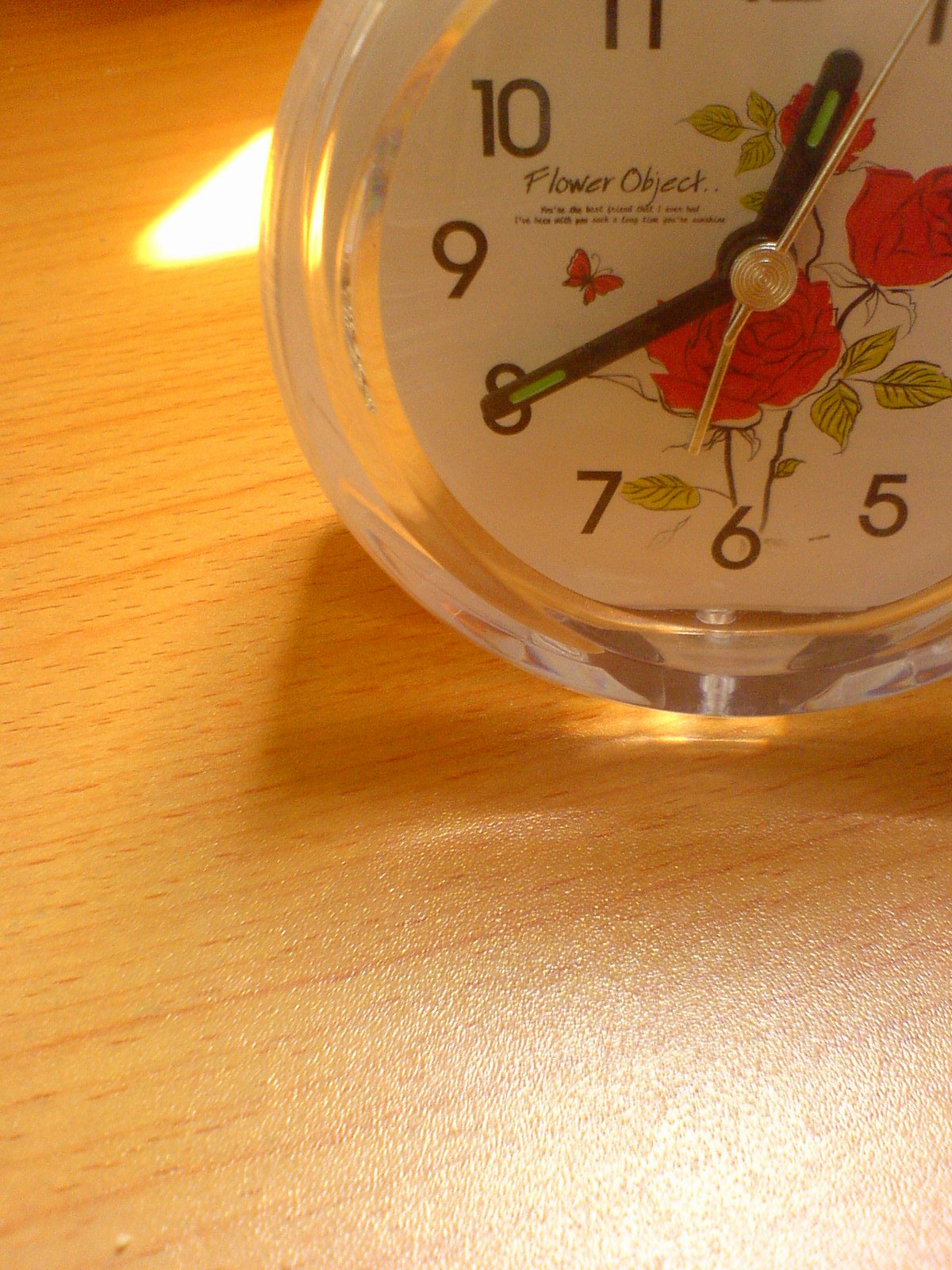The image depicts a close-up shot of an ornate clock partially visible in the upper right corner. The clock face, adorned with three red roses encircled by green leaves and a small red butterfly near the center, is set against a white background. The visible numbers are black or dark brown, specifically 5 through 11, with the other numbers obscured by the edge of the photograph. Encasing the clock face is a clear, glass-like material that gives it a refined appearance. The current time shown is twenty minutes to one. The clock sits on a light orangey-amber wood surface with sunlight brightly reflecting onto it, creating a prominent glare. The hour and second hands are silver, while the minute hand is black. Additionally, there are a couple of light green luminescent indicators that glow in the dark. However, significant portions of the clock are cut off, limiting the view of its full design and structure.